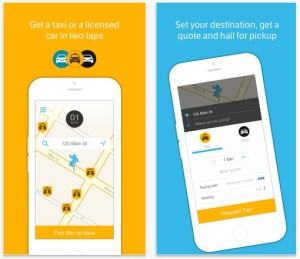This image is a composite of two screenshots, meticulously arranged side by side in a square format. The left screenshot features an orange-themed interface that's challenging to read due to its orange text on an orange background. The text reads, "Get a taxi or a licensed car in two taps," suggesting a rideshare or driver service. A white, digitally illustrated smartphone is prominently displayed, depicting what appears to be a map on its screen.

On the right, the blue-themed screenshot also suffers from readability issues with light blue text on a blue backdrop. It reads, "Set your destination, get a quote, and hail for pickup," further indicating the image’s relevance to a taxi or rideshare service. Similarly, a white digital representation of a smartphone is featured, this time leaning slightly to the left. The interface on this phone includes a prominent yellow button and a black button.

Overall, the image aims to visually communicate the ease and functionality of a digital rideshare service.